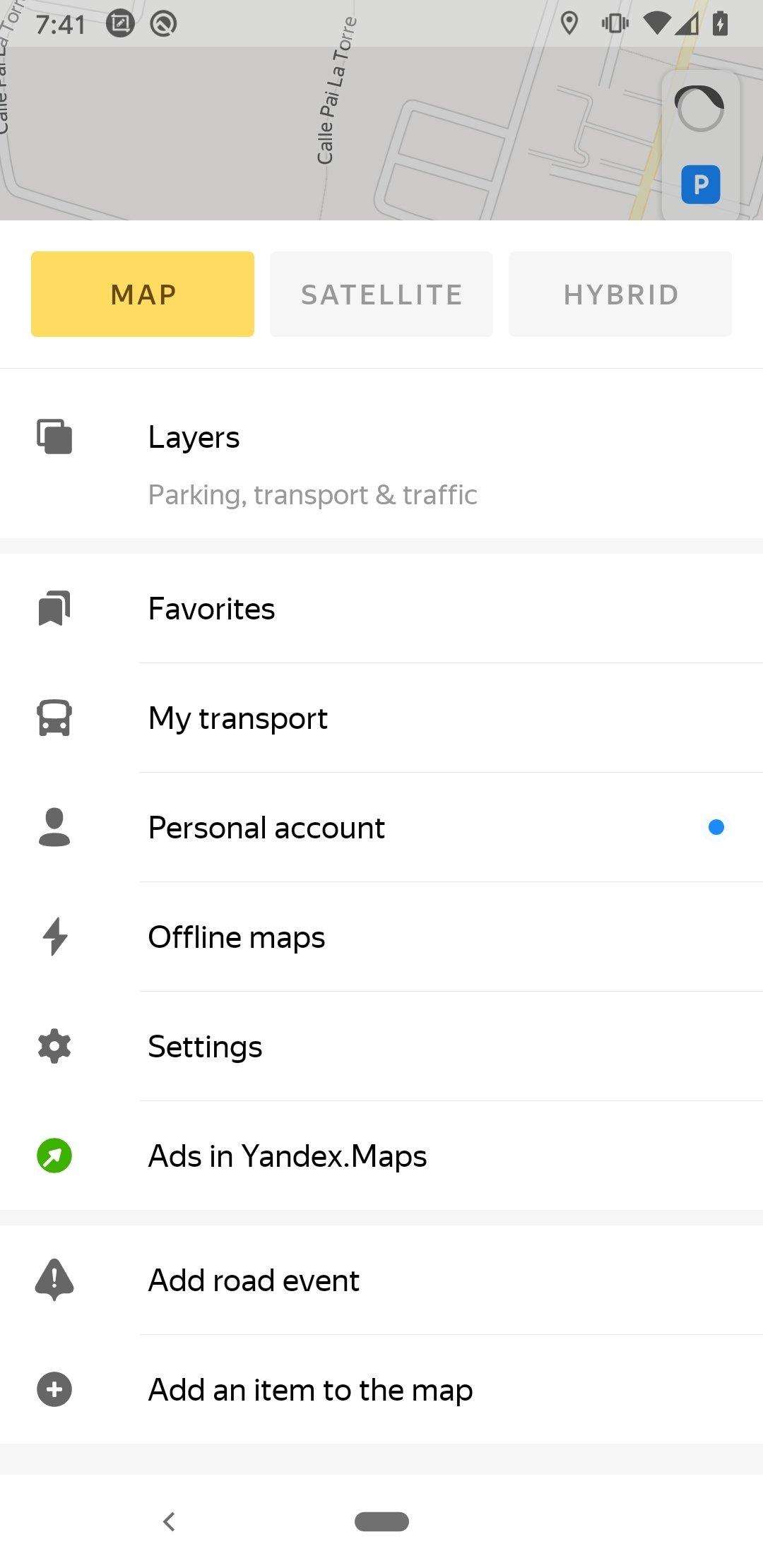Detailed Caption:

In this image, we see a vertically-oriented screenshot of a cell phone screen with a height approximately three times its width. At the top left corner, the time is displayed as 7:41, followed by two icons. On the upper right side, there are five small icons indicating various statuses: wireless signal strength, mobile signal strength, battery life, and others.

Covering the top 20% of the screen, there is a map displayed in a top-down view, typical of what you would see in a navigation app. The map shows a few roads but no significant landmarks.

Below the map, there are three buttons labeled "Map," "Satellite," and "Hybrid." The "Map" button, highlighted with a yellow background and black text, stands out, while the other two buttons are in light gray with dark gray text.

Along the left side of the screen, there is a menu with several icons and labels:
1. The first icon depicts two overlapping pages labeled "Layers."
2. Below that, a section in gray text lists "Parking," "Transport," and "Traffic."
3. Further down is another icon with two overlapping pages featuring a triangular indent at the bottom corner, labeled "Favorites."
4. The next line includes a bus icon labeled "My Transport."
5. Following that is a person icon labeled "Personal Account," with a blue dot to its right.
6. Below that is a lightning bolt icon labeled "Offline Maps."
7. At the bottom, there is a gear icon labeled "Settings."

Each element is neatly arranged, providing a clear and organized interface for the user.